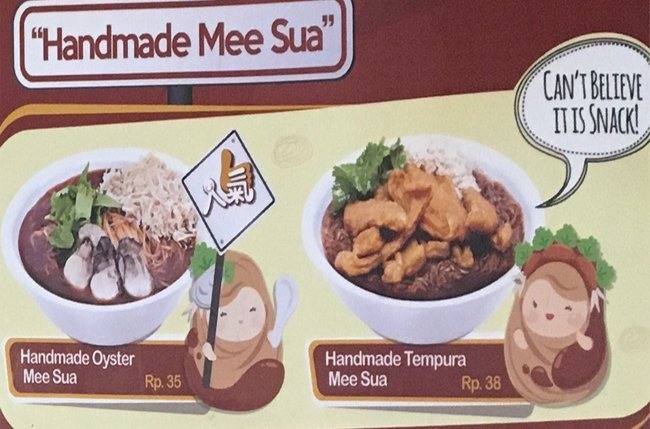This is a detailed picture of a banner or pamphlet advertising two different food items. At the top, it features a white horizontal box with a brown background and inner border, which prominently displays the text "Handmade Misua." Below this, the banner showcases two bowls of beautifully prepared noodle dishes against a cream-colored background. On the left, there is a photo of "Handmade Oyster Misua" priced at RP35, accompanied by an animated character holding up a sign. On the right, there's an image of "Handmade Tempura Misua" priced at RP38, with another animated character next to it, exclaiming in a thought bubble, "Can't believe it is a snack!" Overall, the menu utilizes a color palette dominated by brown and yellow tones, with both photographs and charming animated characters enhancing the visual appeal of the advertised snack noodle bowls.